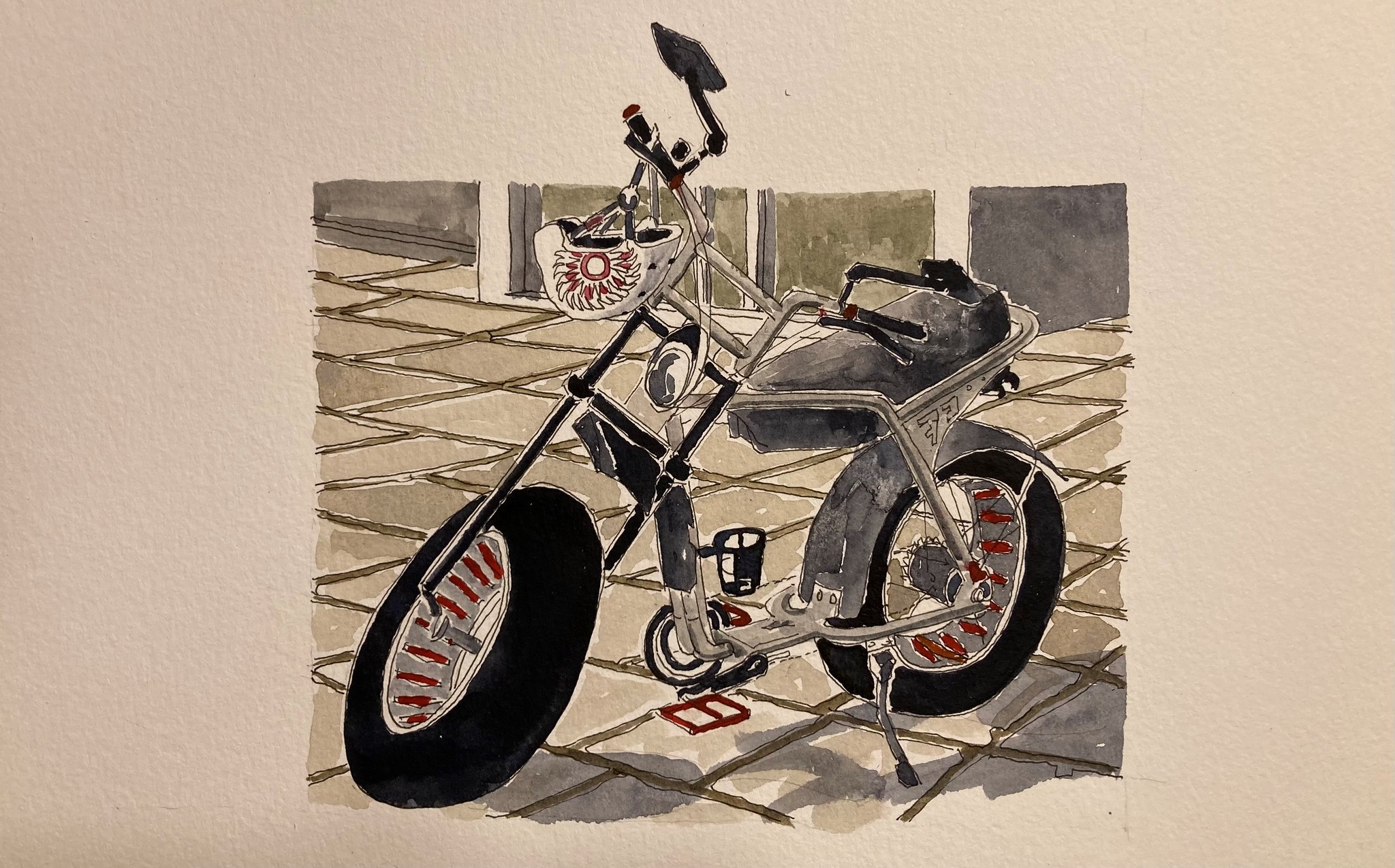The image is a detailed watercolor painting on a white paper sheet, depicting a parked motorcycle that resembles a Harley. The motorcycle is positioned inside a rectangular frame, with its large wheels extending beyond the rectangle. The bike is oriented towards the right, with the front wheel turned slightly downward. It features a grey and black frame, with the seating cushions, back fender plate, and front wheel frame all in grey. Red accents adorn the rims, and both black handlebars are equipped with red and black mirrors.

A white helmet with a red and white sunray design hangs from the top of the handlebars, dangling downward. The bike also has a pair of mudguards, a large, wide seat suitable for two people, and a kickstand supporting it on the ground. Additionally, there is a cup holder attached to the frame. The floor beneath the motorcycle is made of grey and brown square tiles, adding a textured background to the illustration.